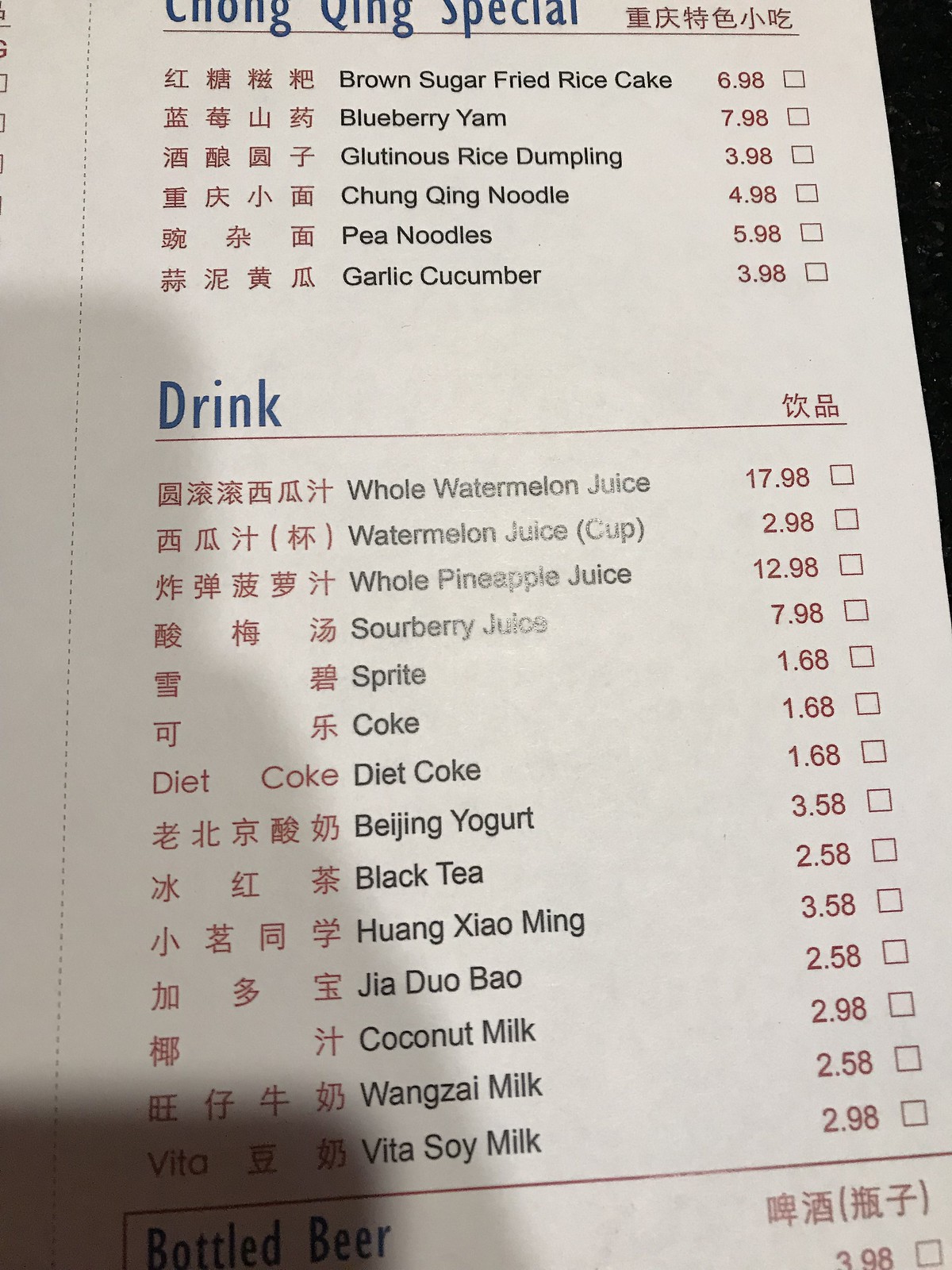A photograph of the last page of a Chinese food menu, featuring a crisp white background. The menu's headings are elegantly printed in blue text, providing a striking contrast to the rest of the content. Each item description on the menu is meticulously written in traditional black Chinese characters, while the prices stand out in vivid red. 

The upper section of the menu is dedicated to "Chongqing Specials," offering an enticing selection of dishes such as Brown Sugar Fried Rice Cake, Blueberry Yam, Glutinous Rice Dumpling, Chongqing Noodle, Pea Noodles, and Garlic Cucumber. 

Below the special dishes, there is a comprehensive drinks section that lists refreshing beverages including Whole Watermelon Juice, Watermelon Juice in a Cup, Whole Pineapple Juice, Sour Berry Juice, a wide assortment of soft drinks, Beijing Yogurt, Black Tea, Coconut Milk, Wangzai Milk, and Vitasoy Milk.

At the bottom of this page, there appears to be a category designated for bottled beers. However, the image is cut off at this point, leaving the specific types of beers offered out of view.